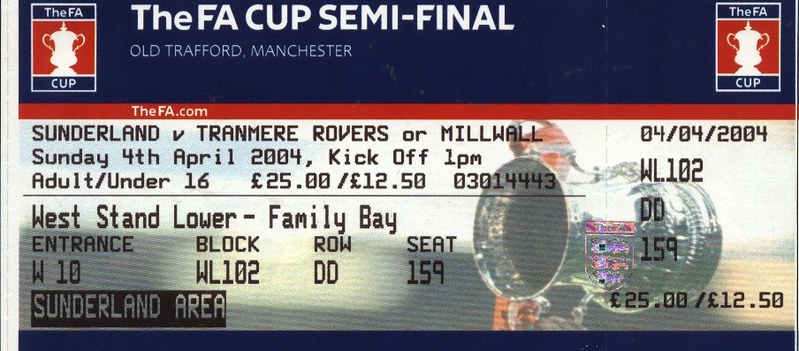The ticket for the FA Cup Semi-Final features a dark blue header with the text "THE FA CUP SEMI-FINAL" prominently displayed in large white font. Beneath this, in small all-caps font, it reads "Old Trafford, Manchester." A red bar follows, displaying "thefa.com" in white text, flanked on either side by white trophy icons within red boxes. Below this, in black font, it states the match details: "Sunderland vs. Tranmere Rovers or Millwall, Sunday 4th April 2004, Kickoff 1 p.m." The ticket specifics include "Adult £25 / Under 16 £12.50," and a reference number "03014443." The bottom section of the ticket also features a visual, likely of someone raising the cup, with text overlaying the image. Additional information notes that this ticket is for the West Stand Lower, Family Bay, Sunderland area.